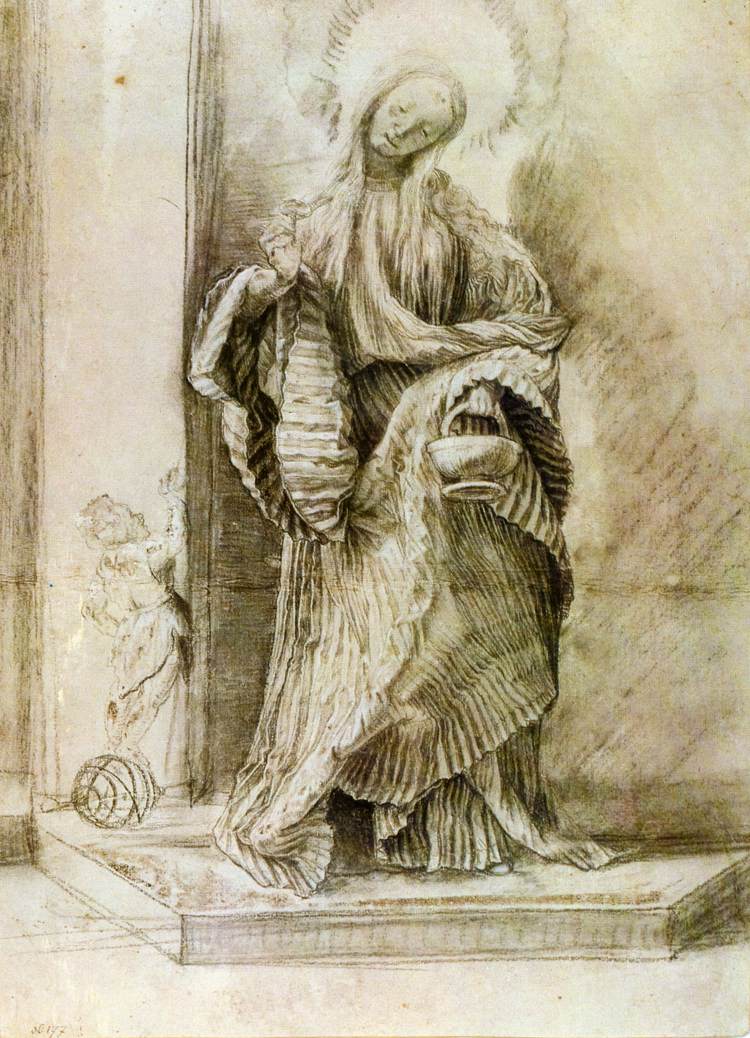The image is a black, white, and sepia-tone drawing with a detailed, almost ethereal quality that combinine elements of medieval religious art and modern geometric patterns. At the center of the composition stands a woman with long, flowing hair extending past her shoulders. Her head is gently tilted to the side, adding to the serene and contemplative atmosphere of the piece. She appears to have a faint halo surrounding her head, evoking an image reminiscent of the Virgin Mary.

She is wearing a voluminous, draped robe adorned with intricate, geometric pleats that cascade down her form, giving it a balanced blend of fluidity and structure. The garments have a faded, textured quality, achieved through blending techniques that suggest pen and ink or graphite rendering. Each fold and stripe of the robe is meticulously detailed, with rough edges adding to the vintage feel of the artwork.

Her right hand is raised and extended outward, while her left hand holds a basket or pedestal-like object, its base standing out with notable prominence. In the background, a small figure stands in a doorway with one foot on what appears to be a ball, adding another layer of depth to the scene.

Overall, the artwork exudes a calm, almost sacred presence with impressive attention to detail in both the figure's appearance and the surrounding elements. The absence of text and the monochromatic yet slightly sepia color palette contribute to the timeless, contemplative quality of this modern yet historically inspired piece.